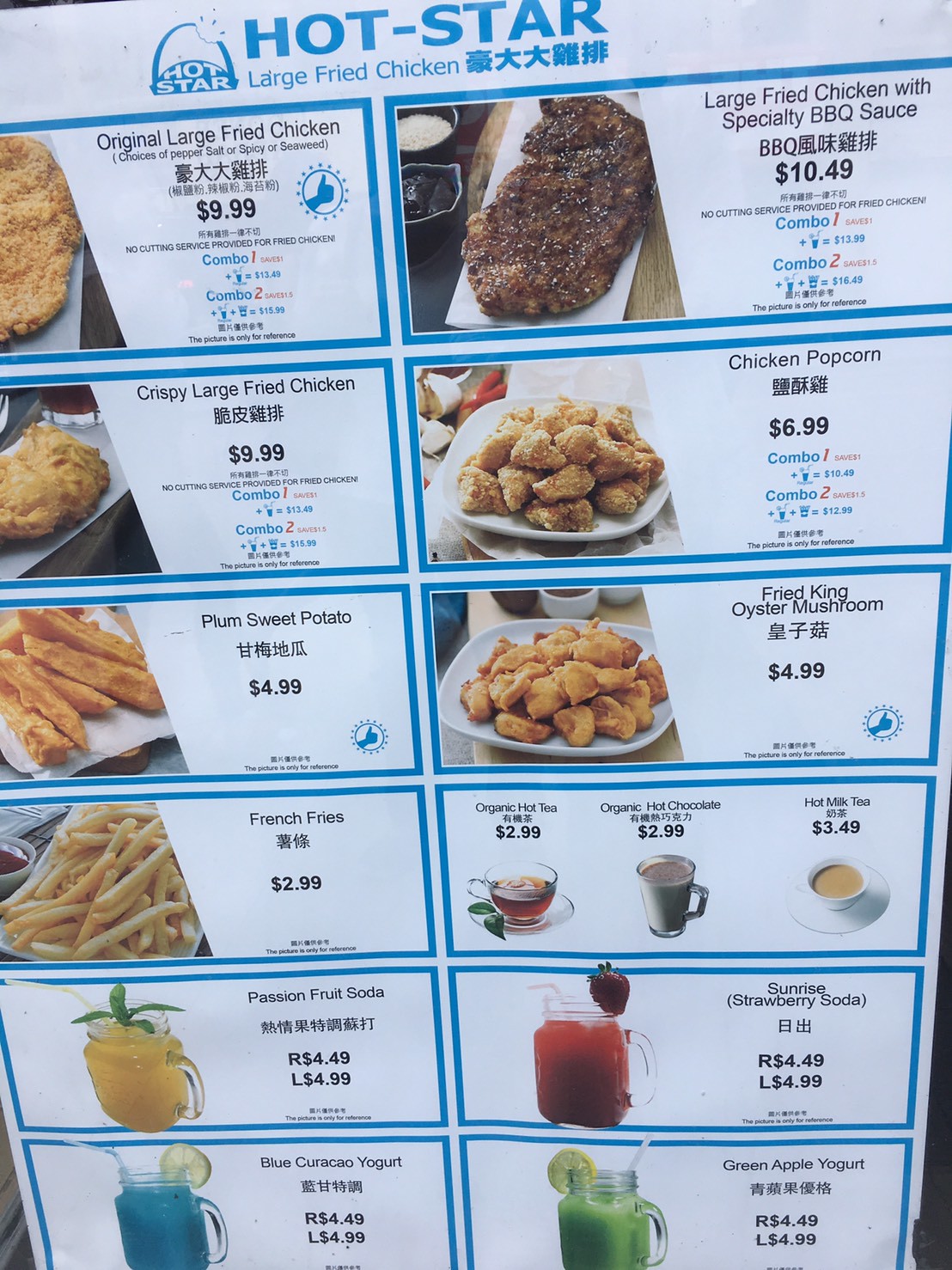This photograph showcases a restaurant menu elegantly designed with a white background adorned with horizontal blue rectangles. Inside each blue-bordered rectangle, menu items are listed with accompanying photographs, names, and prices. The text is presented in both English and an unidentified Asian language. 

Prominently featured at the top of the menu are the words "Hot Star Large Fried Chicken" along with Asian characters. On the left side, the Hot Star logo, which resembles a taco with a bite taken out of it, reinforces the branding.

The right-hand side lists the items as follows:

1. **Large Fried Chicken with Specialty BBQ Sauce - $10.49**: Notably, the image seems to display a steak rather than chicken.
2. **Chicken Popcorn - $6.99**
3. **Fried King Oyster Mushroom - $4.99**
4. **Beverages** (housed within a single rectangle):
    - Organic Hot Tea
    - Organic Hot Chocolate
    - Hot Milk Tea
5. **Sunrise Strawberry Soda**
6. **Green Apple Yogurt**

On the left-hand side, from the top:

1. **Original Large Fried Chicken - $9.99**: Customers can choose between Pepper Salt, Spicy, or Seaweed flavors.
2. **Crispy Large Fried Chicken - $9.99**
3. **Plum Sweet Potato - $4.99**
4. **French Fries - $2.99**
5. **Passion Fruit Soda**
6. **Blue Curacao Yogurt**

The bottom portion of the menu is not visible in the photograph, suggesting additional items extend beyond the captured image. 

This detailed menu layout offers a mix of savory fried chicken options, side dishes, and both hot and cold beverages, catering to various tastes.